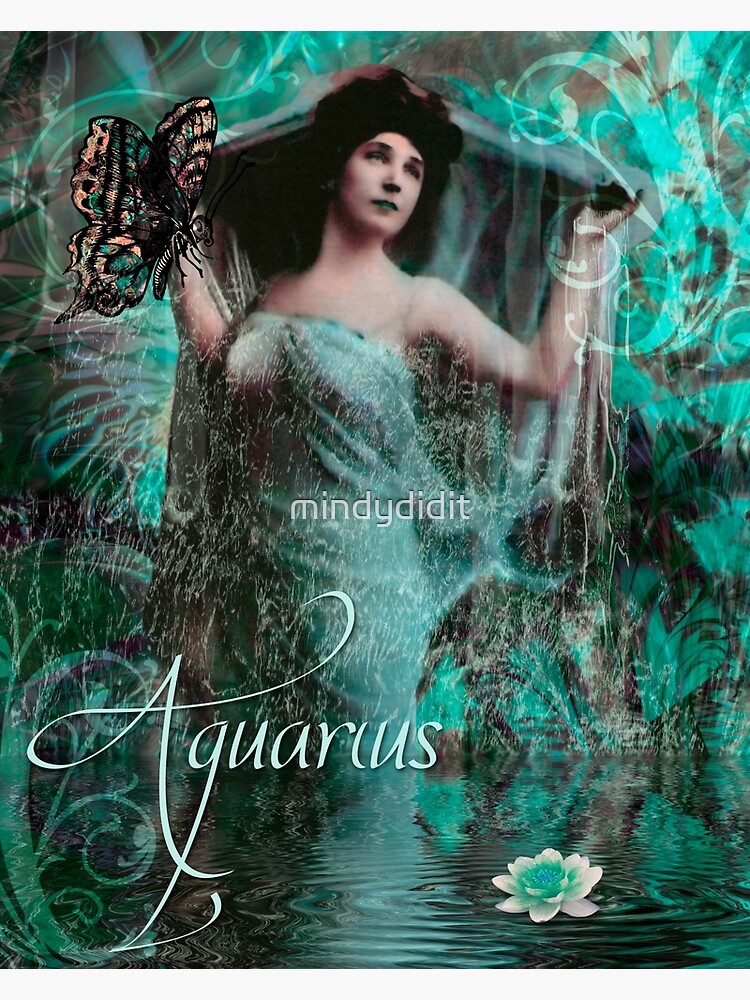The image appears to be a digitally created, vertically oriented Art Deco-style poster or book cover. It features a central pale, cherubic woman with black curly hair, reminiscent of Renaissance figures. She is standing in a clear, rippling lake, with teal and gray mist-like tendrils rising from the water, and a green and white lotus flower floating at the bottom left.

The woman is wearing a strapless teal dress and holds a diaphanous veil above her head with outstretched arms, their movements creating an illusion of flow and grace. In her right hand, she holds a large, colorful butterfly in shades of black, peach, orange, and green, while her left hand grasps an unidentified black object. The word "Aquarius" is spelled out on the bottom right in light teal script, and a watermark reading "Mindy did it" appears centrally in white.

Overall, the image is a harmonious blend of teal, green, and white, with abstract swirling patterns and floral motifs that enhance its ethereal, water-themed ambiance.